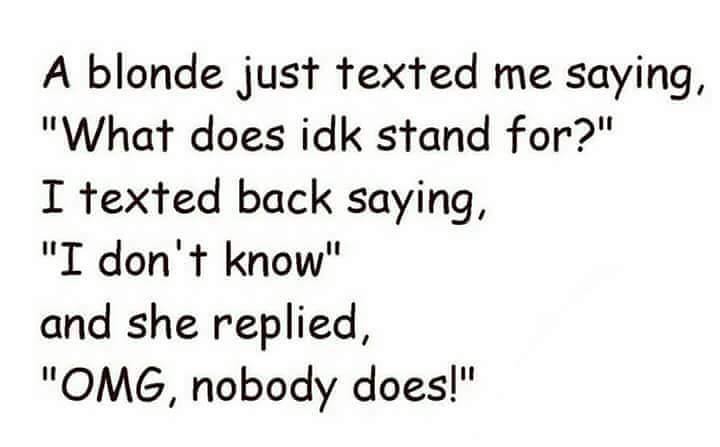This image features a humorous text-based joke printed in black letters on a completely white background. The joke reads: "A blonde just texted me saying, 'What does IDK stand for?' I texted back, 'I don't know.' She replied, 'OMG, nobody does!'" The text is left-aligned and straightforward, likely printed on a standard piece of paper. The image contains no additional graphics or framing elements, and is simply a play on the misunderstanding of the abbreviation "IDK," which stands for "I don't know."